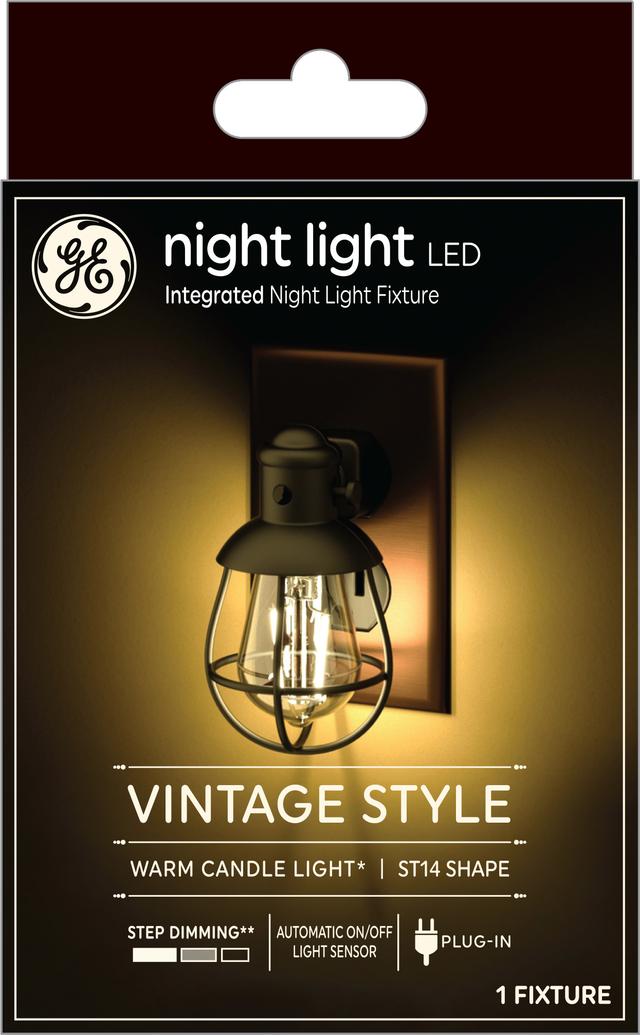The image depicts the packaging of a GE Nightlight, featuring an LED integrated nightlight fixture with a vintage lantern design. The packaging, designed to be hung on a store display, showcases a visibly illuminated nightlight emitting warm, candle-like light through a glass bulb encased in a metal cage, resembling an old-fashioned lantern. The package background is a dark brown, almost black, with detailed text explaining the product's features, including step dimming and an automatic on-off light sensor. Prominently displayed is the white GE logo, signifying its manufacture by General Electric, reassuring of its quality. The light is shown plugged into a copper switch plate, casting a gentle glow on the wall behind it. The model number, ST-14, is also indicated, emphasizing its vintage style and modern functionality.